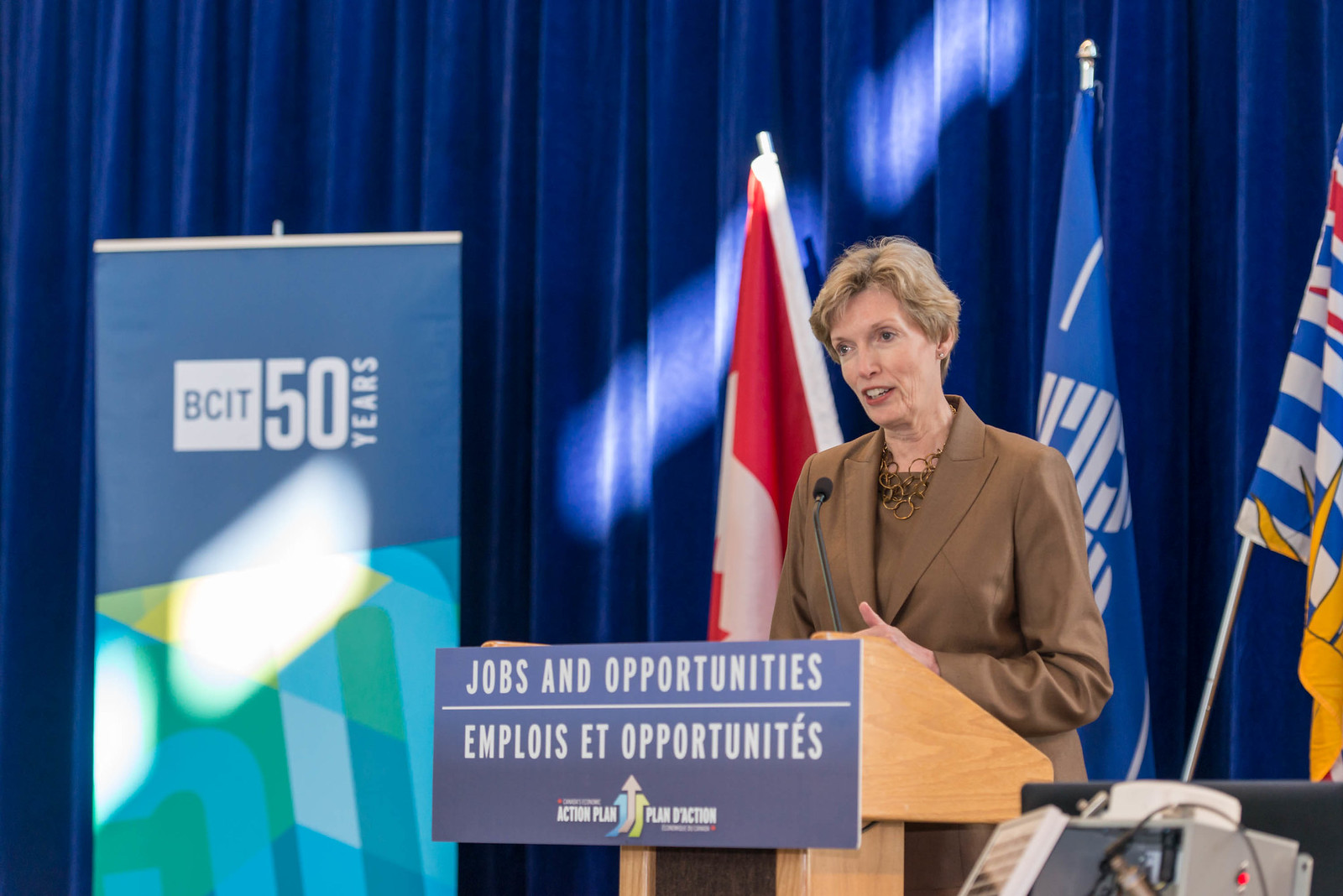The image shows a woman with short, blondish-brown hair and wearing a monochrome brown suit, consisting of a jacket and blouse, standing at a wooden podium. She appears to be in her late 60s and is speaking into a thin microphone positioned up towards her face, with her hands held out in front of her as she talks. The podium features a blue rectangular sign with white lettering that reads "Jobs and Opportunities," repeated below in a different language, accompanied by a logo.

Behind her, large, dark blue theater-type curtains serve as a backdrop. To her left, there is a banner on an easel stating "BCIT 50 years." Additionally, you can see three flags, one of which is identified as the American flag, while the others appear to be representing different countries with their distinctive red and white, blue and white, and red, white, and blue with yellow patterns. The sun is shining through windows, causing some glares across the curtains and one of the signs.